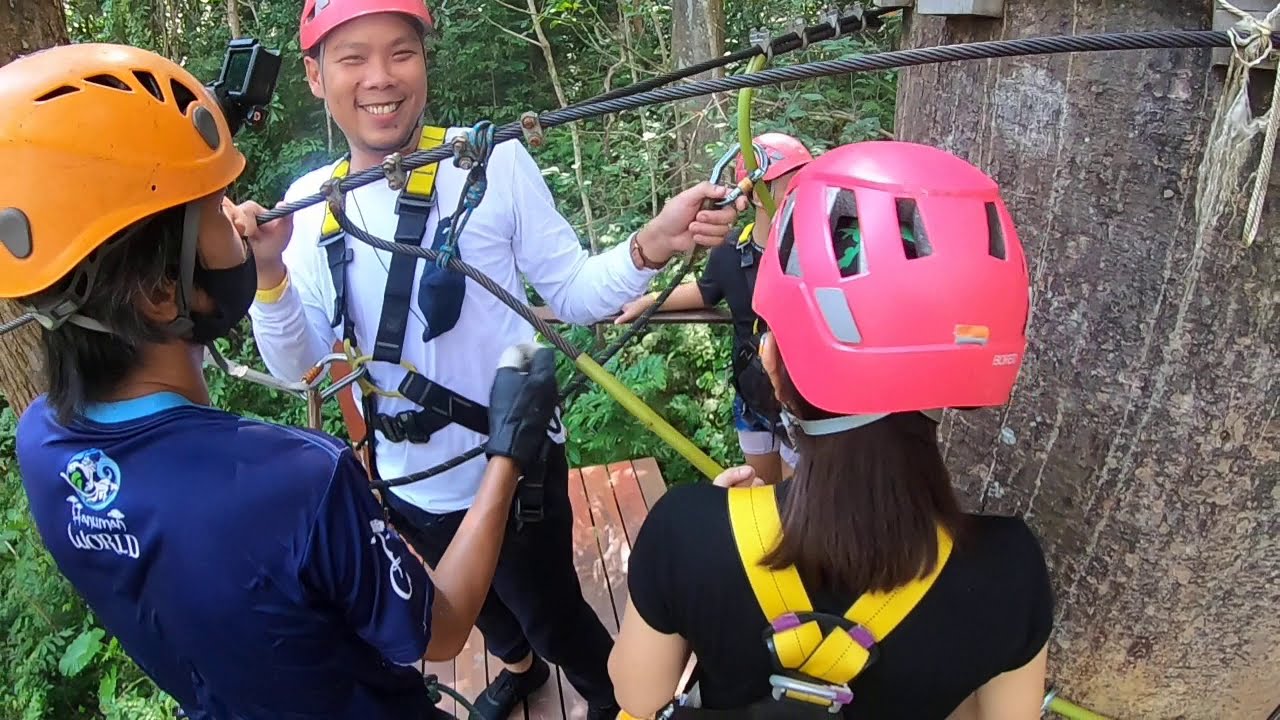In this vibrant and energetic image, a group of four Asian individuals, likely Filipino, are preparing for an exhilarating zipline adventure in a lush, dense forest. The focal point of the image is a young man in his early twenties, smiling directly at the camera while fastening his harness onto the zipline cable. Dressed in a long-sleeved white shirt, black pants, and a pink safety helmet, he exudes excitement and readiness. The surrounding greenery and the sturdy tree to his right set a picturesque backdrop, indicating their elevated position on a platform. To his left, we see another person in an orange helmet and a blue jersey, seemingly assessing the zipline clip the smiling man holds. Further right, a woman with long brown hair wearing a pink helmet attentively looks on. All three appear to be deeply engrossed in their upcoming adventure, their faces turned away from the camera. A fourth person, partially obscured, adds to the bustling energy of the image. The scene captures a moment of eager anticipation and teamwork amid the natural beauty of the probable Asian jungle setting.